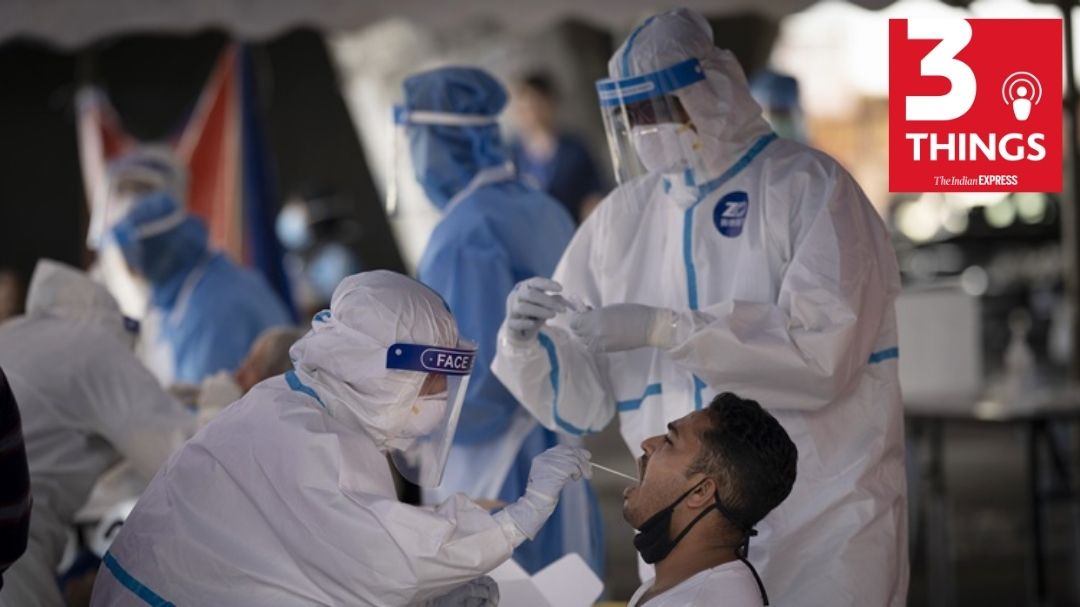In the screenshot, a man is undergoing a COVID-19 test. He has his mask pulled down to his chin while a healthcare worker in full protective gear, including a white jumpsuit, gloves, head covering, and face shield, uses a swab to collect a sample from his mouth. Another healthcare worker, similarly attired, holds the testing materials. In the dimly lit background, additional medical personnel are visible, also conducting tests. Several tents are set up, indicating a larger testing site. To the right of the central figures is a table with a green sign displaying the number "3" in white, alongside text that says "Express" and other, less legible words.